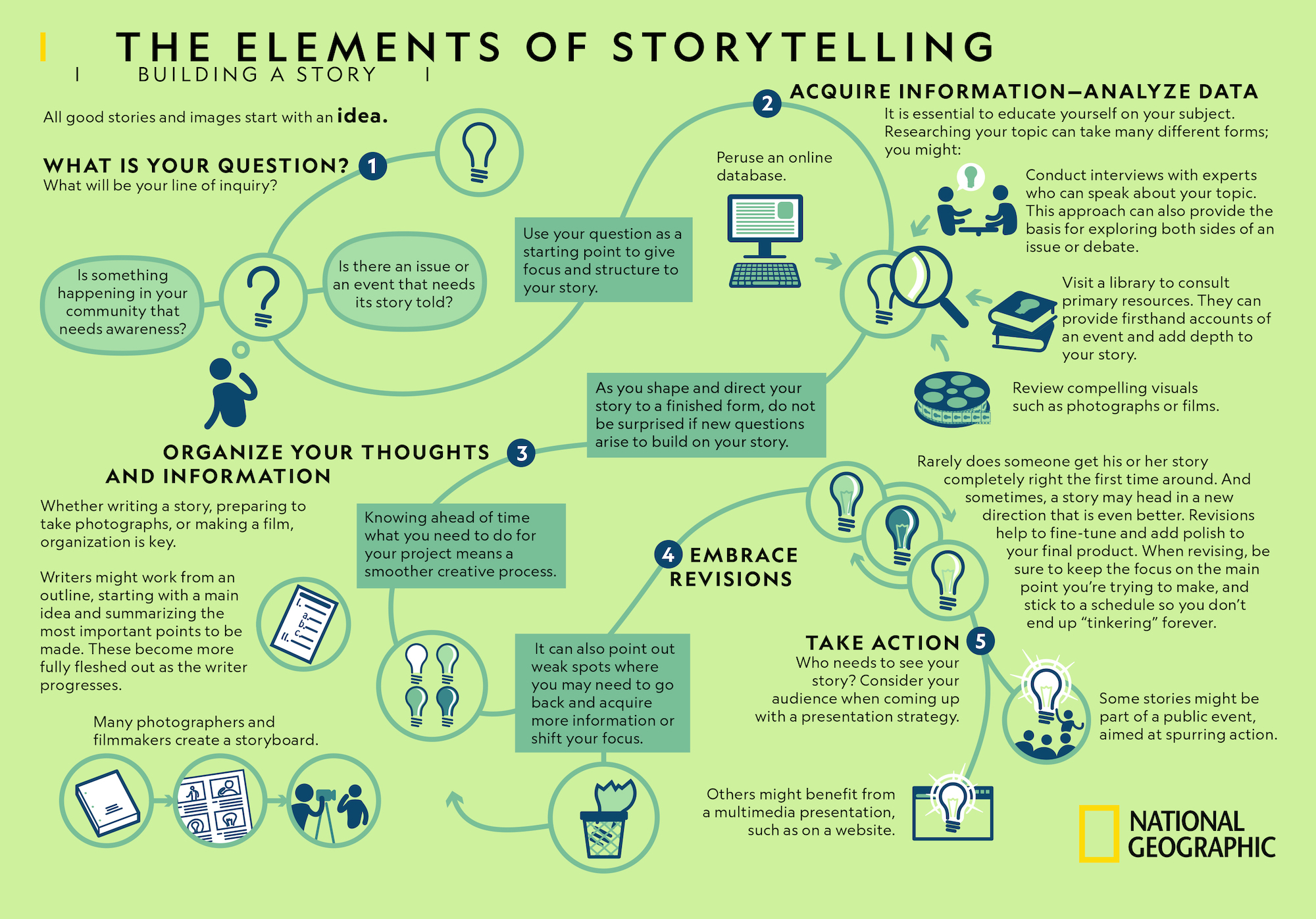The image is a detailed, illustrated chart from National Geographic, with a light lime-green background and a title in bold black letters at the top that reads "The Elements of Storytelling." Below it, in smaller font, the subtitle "Building a Story" is displayed. The bottom right-hand corner features the iconic yellow rectangle logo of National Geographic, accompanied by the text "National Geographic" in black capital letters. 

Starting from the top of the page, a thin blue line winds down like a path with various twists and turns, marking five key points in the storytelling process. Each point is distinguished by a number within a colored circle, accompanied by small paragraphs of instructional text and relevant icons. 

- **Point 1:** Represented by a light bulb icon within a circle and the text "What is your question? What will be your line of inquiry?" This encourages identifying a focal question for your story, emphasizing the importance of asking questions to highlight community needs, issues, or events.
- **Point 2:** "Acquire information / Analyze data," which stresses the collection and analysis of relevant data and poses additional probing questions.
- **Point 3:** "Organize your thoughts and information," focusing on structuring the collected data and ideas logically.
- **Point 4:** "Embrace revisions," highlighting the necessity of refining your story through multiple iterations.
- **Point 5:** "Take action," the final step prompting the storyteller to implement their narrative effectively.

Overall, the chart provides a comprehensive guide to crafting a well-structured and impactful story, visually leading the viewer through each essential step in the process.